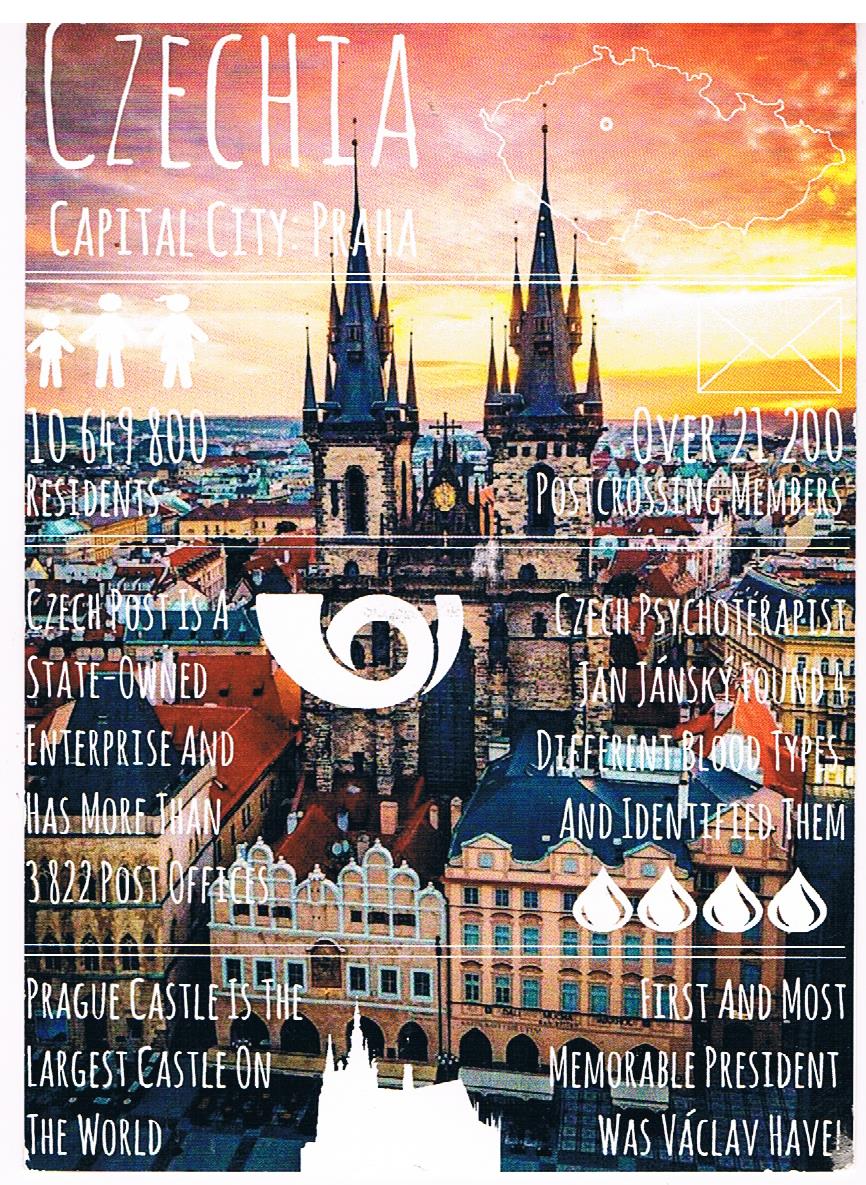The image depicts a vibrant poster highlighting key details and landmarks of Czechia, with a prominent mention of its capital city, Praha (Prague), in white text at the top. Central to the image is a picturesque portrayal of the city, featuring a large, imposing cathedral flanked by numerous multi-colored buildings with green windows. The skyline glows with warm orange and yellow hues, creating a striking backdrop. The poster also provides various interesting facts, including the population of 10,649,800, the presence of over 21,200 post-crossing members, and mentions of state-owned Czech Post with its 3,822 post offices. Further highlighted are historical and cultural points, such as Prague Castle, known as the largest castle in the world, and the contributions of Czech psychotherapist Jan Jansky, who identified different blood types. Lastly, the poster commemorates Václav Havel as the first and most memorable president. Various logos, including one resembling restroom signage, add to the eclectic, informative nature of the design.